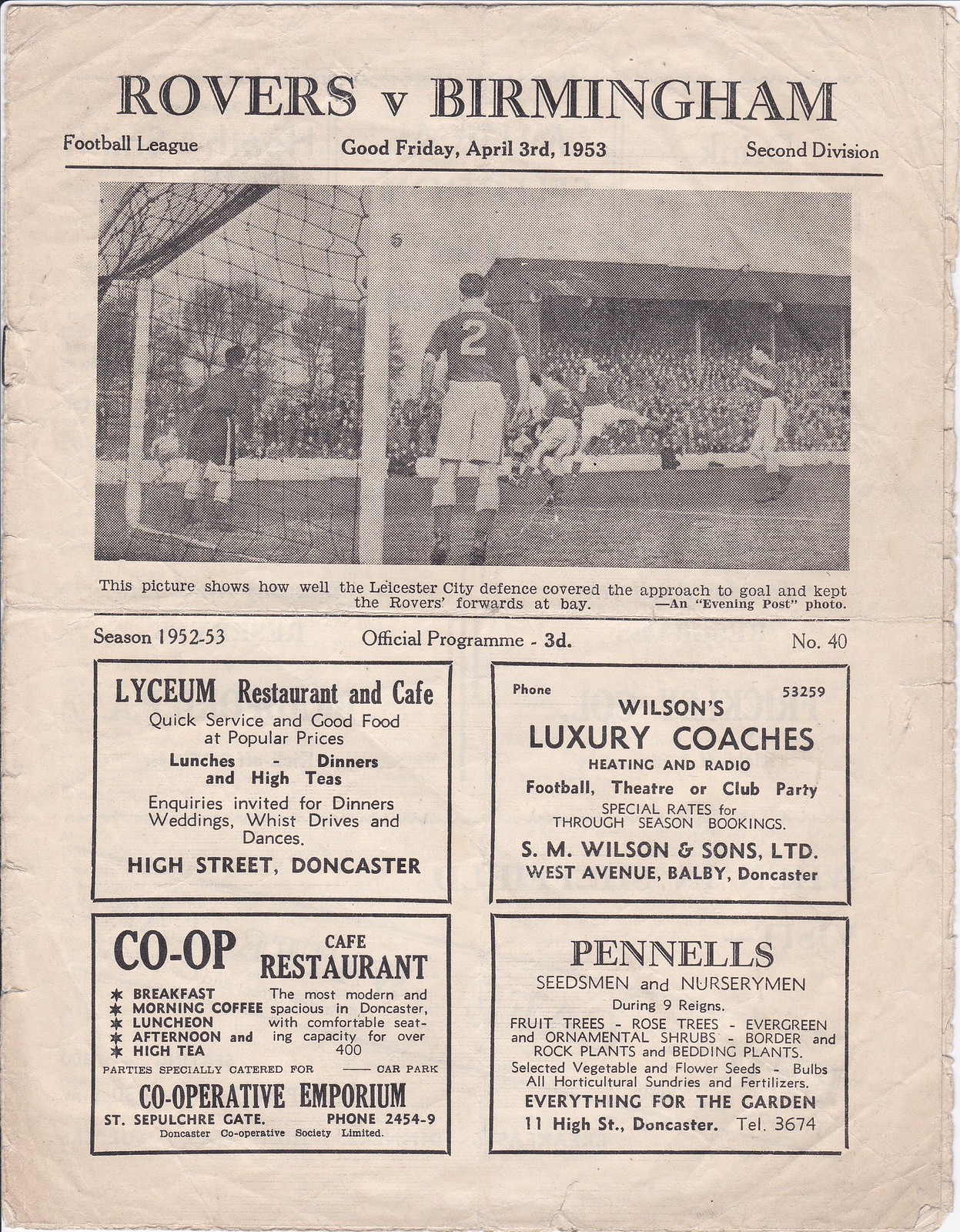This detailed caption provides a comprehensive view of a 1953 football program:

The football program, dated Good Friday, April 3, 1953, showcases the match between Rovers and Birmingham in the Second Division of the Football League. The aged, slightly wrinkled cover features a black and white photograph prominently placed beneath the heading "Rovers vs. Birmingham", highlighting Leicester City’s defense effectively thwarting the Rovers' forwards. The main image captures soccer players in action, focusing on a player with the number two on his shirt standing near the goal, with spectators visible in the stadium background. The caption beneath the photo, credited as an Evening Post photo, reads: "This picture shows how well the Leicester City defense covered the approach to goal and kept the Rovers forwards at bay." 

The title panel further specifies this as the official program (number 40) for the 1952-53 season. Below the photo, there are four distinct advertisements: 

1. **Lyceum Restaurant and Cafe** - Promoting quick service with good food, offering lunches, dinners, high teas, as well as arrangements for events such as weddings and dances, located on High Street, Doncaster.
2. **Wilson's Luxury Coaches** - Featuring heated and radio-equipped coaches available for football, theater, or club parties, with special rates for season bookings; located at West Avenue, Balby, Doncaster.
3. **Co-op Cafe Restaurant** - Billed as the most modern and spacious in Doncaster, with seating for over 400 patrons and catering for various meals and parties, situated at the Cooperative Emporium, St. Sepulchre Gate.
4. **Pinnell Seedsmen and Nurserymen** - Offering a wide range of gardening supplies including fruit trees, rose trees, various plants, seeds, and horticultural sundries, located at 11 High Street, Doncaster.

All text on the page is presented in black, contributing to the historic and classic feel of this well-preserved football program.